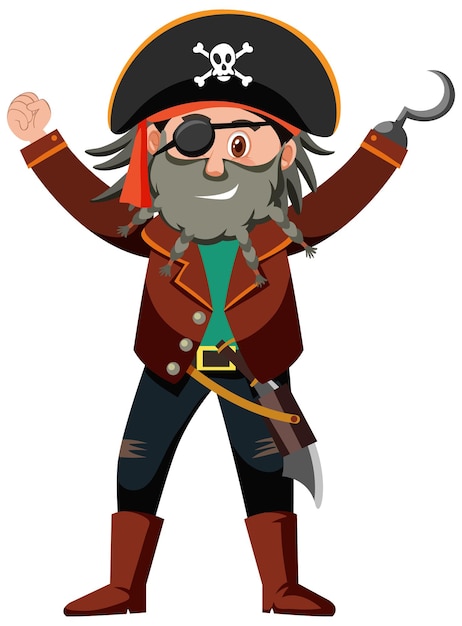This detailed digital vector illustration depicts a cheerful pirate with both arms raised in a V shape, reminiscent of the YMCA dance. He sports a large black pirate hat adorned with a skull and crossbones. From beneath the hat, long gray hair and a bushy gray beard flow out. A black eye patch covers his right eye, while his visible brown eye twinkles with a friendly smile.

The pirate is dressed in a rugged, brown jacket embellished with orange details, under which he wears a blue-green shirt. A sturdy brown belt with a prominent yellow buckle secures his ensemble. Further adding to his pirate persona, he carries a machete or hatchet at his side, fastened to his belt.

His pants are primarily black with the top portion being blue, and they are accompanied by brownish-orange boots. Notably, his left arm ends in a silver or metal hook, replacing his hand. The overall impression is of a friendly pirate, enjoying a moment of triumph or joy, as his lively pose and beaming expression suggest.